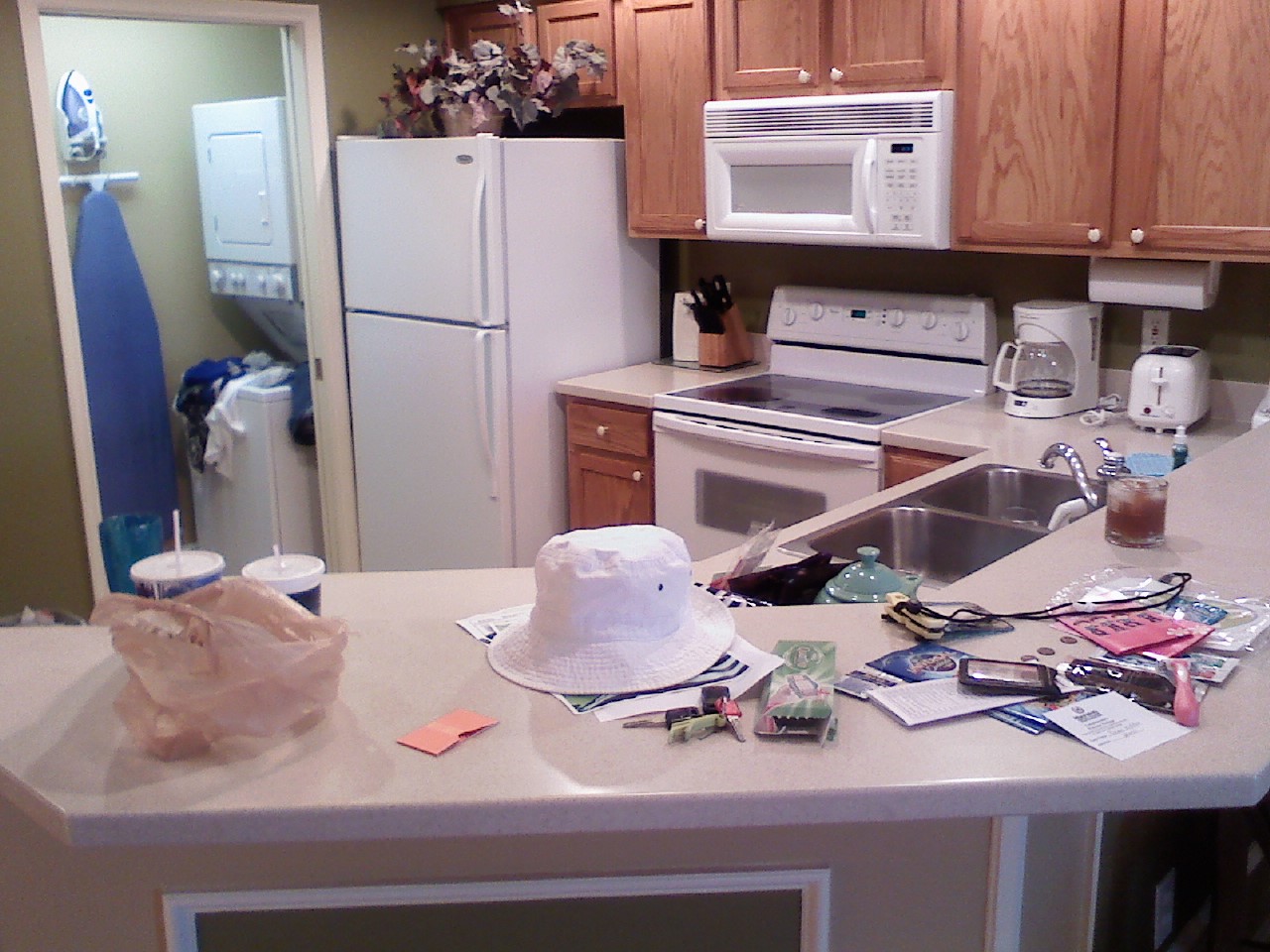This photograph captures a bustling kitchen that appears to have been actively used throughout the day, evident from the considerable mess strewn across the front. Dominating the foreground is a counter shaped like a boomerang, creating a sweeping curve from one side of the kitchen to the other in a C or D shape. On the left side of the counter, there are two dark blue cups with straws, hinting that the occupants might have brought drinks from a restaurant. Nestled next to these cups is a brown bag, presumably from takeout.

Central to the counter is a white hat that at first glance resembles a cake. The surface is cluttered with various items, including some unidentifiable objects, a hook, and something pink. Further back, the kitchen reveals essential appliances: a silver-colored sink, a white oven, stove, and microwave. The microwave is integrated just below the brown cabinets, making it a permanent fixture. To the top right, a white coffee maker and a white toaster can be spotted, adding to the array of kitchen gadgets. The brown cabinetry above the microwave provides additional storage space, contributing to the kitchen's overall functionality amidst the chaos.